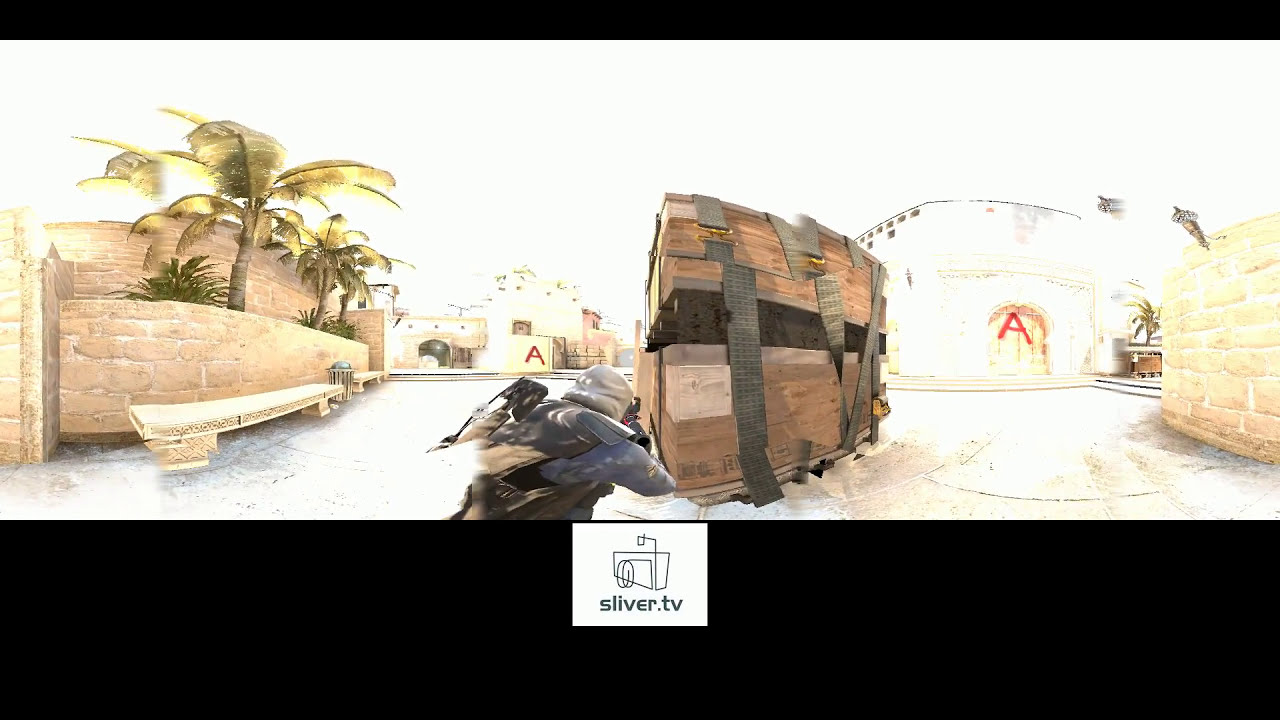The image is a highly detailed still frame from a video game, likely presented by Sliver TV, as indicated by the logo at the bottom center of the image. The logo features a white rectangle with a rough, scribbled drawing of a building with a streetlight, followed by the text "sliver.tv."

The central focus of the image is a street scene, possibly set in an Arab country. The overall background is predominantly white, fading into a series of structures adorned with large, painted letters "A." On the far right, a light brown door also bears a large "A," adjacent to a tan-colored brick wall. In the middle ground of the scene stands a stack of two wooden crates, secured by black straps with visible gold clasps, resembling belts more than duct tape. 

Crouching behind the crates is a man clad in tactical gear, including a white hood and what seems to be armor. Though not clearly visible, it appears he is holding a gun, suggesting an urban warfare scenario. To the left of this action, a tan wall emerges, accompanied by a palm tree and a stone bench; between the benches lies a garbage can. This vivid depiction intricately blends elements of tension and realism, framing the man’s cautious advance through a conflict-ridden street.